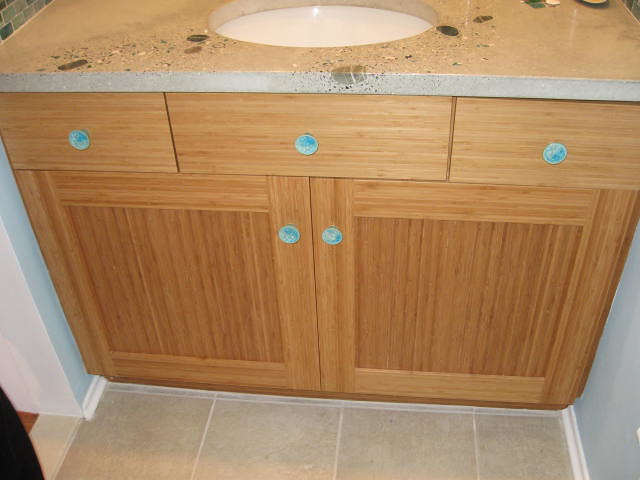The image depicts a bathroom under construction. Dominating the scene are wooden cabinets with contrasting blue caps. The countertop, which appears to be spotted and dirty, awaits final cleaning or installation. The floor is covered in gray tiles, complementing the blue walls on the right and a light blue wall on the left. Visible in the middle of the countertop area are three circular openings, alongside two additional circular openings, likely intended for fixtures yet to be installed. The white basin at the top suggests an incomplete sink setup. The description also mentions white tiles at the top, adding to the bathroom's unfinished aesthetic.